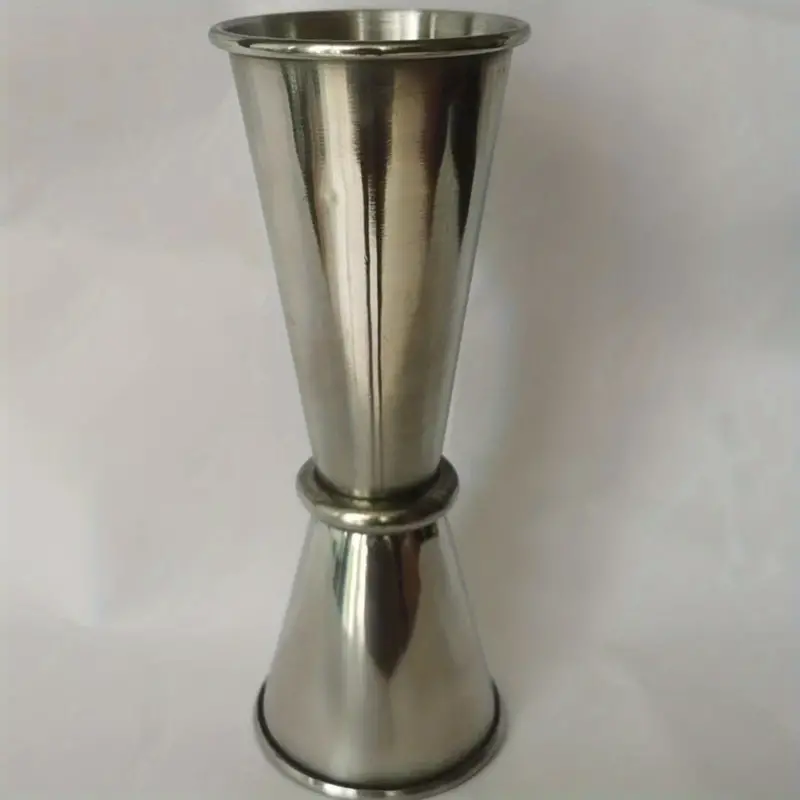This image features a highly reflective silver metal jigger used in bartending, designed for accurately measuring alcohol when mixing drinks. The jigger, placed on a white or light off-white surface, boasts two cone-shaped sides that flare out at the top, each side curved over at the lip. The smaller side likely measures half an ounce while the larger side measures a full ounce, though it may appear deceptively elongated in the photo. A distinctive flared ring separates the two measuring sections, allowing for easy flipping to select the desired measure. The polished, chromed finish produces a mirror-like reflection that subtly distorts the surroundings into abstract shapes and smears of color. The overall design ensures quick and precise pouring, making it an essential tool for any bartender.